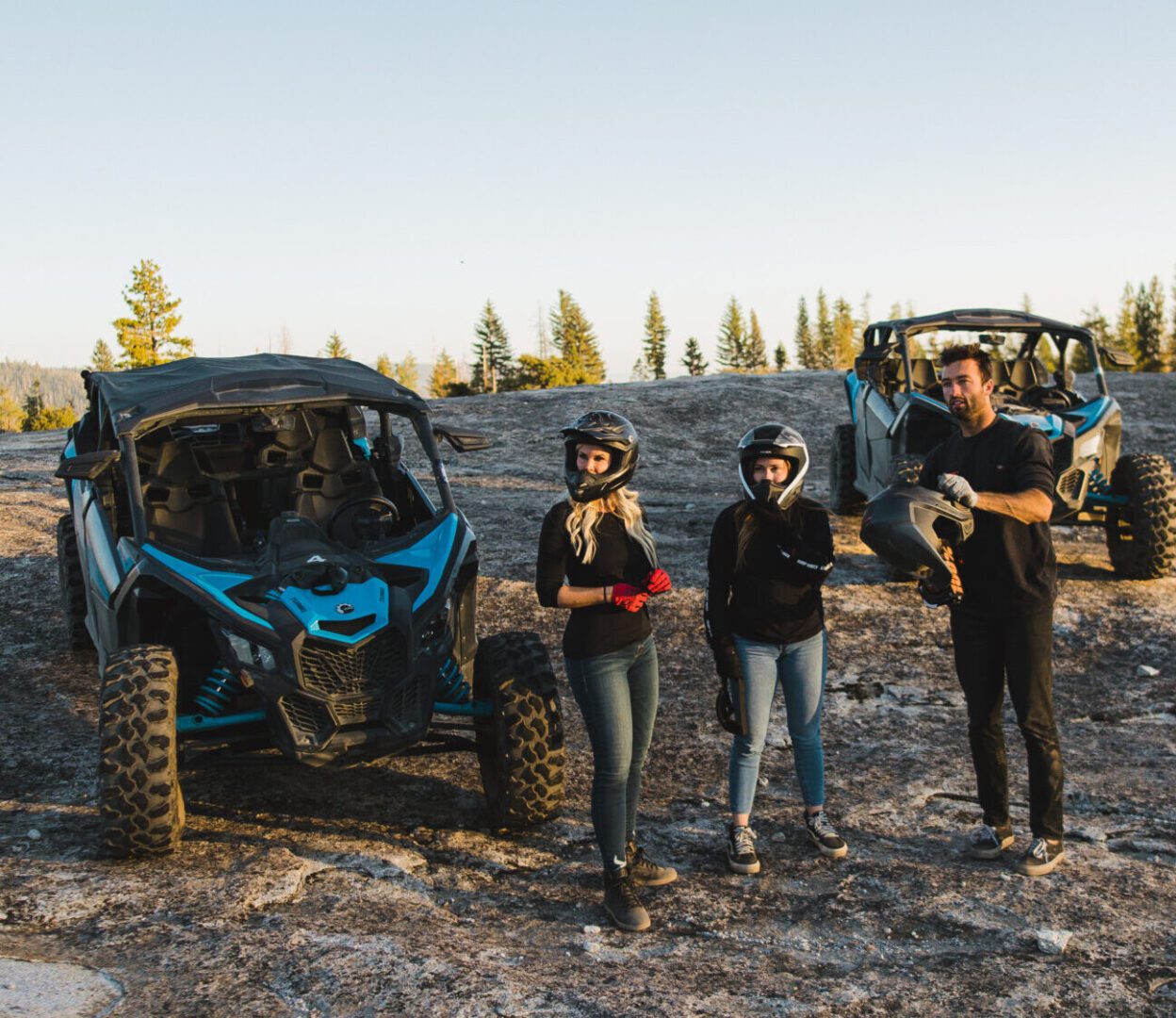A family of three is captured in this vibrant, sunlit image set against the backdrop of a serene, pine-filled landscape. They appear geared up for an off-roading adventure with their blue dune buggies, parked prominently behind them. The father, positioned to the right, is in the process of fastening his helmet, while the mother, standing to the left, is already fully equipped with her helmet and gloves. Her blonde hair peeks out from under her helmet. Between them stands their child, also clad in all the necessary gear, their gaze directed off to the side, absorbed in something beyond the frame. The family is dressed predominantly in black; the women in black tops paired with jeans, and the man in black pants. The two robust dune buggies, featuring convertible-style cloth roofs (one of which is removed), hint at an adventurous spirit ready to tackle the terrain. The setting is alive with the stark contrast of a bright winter day that illuminates the entire scene, casting a beautiful glow over the family and their impressive vehicles.